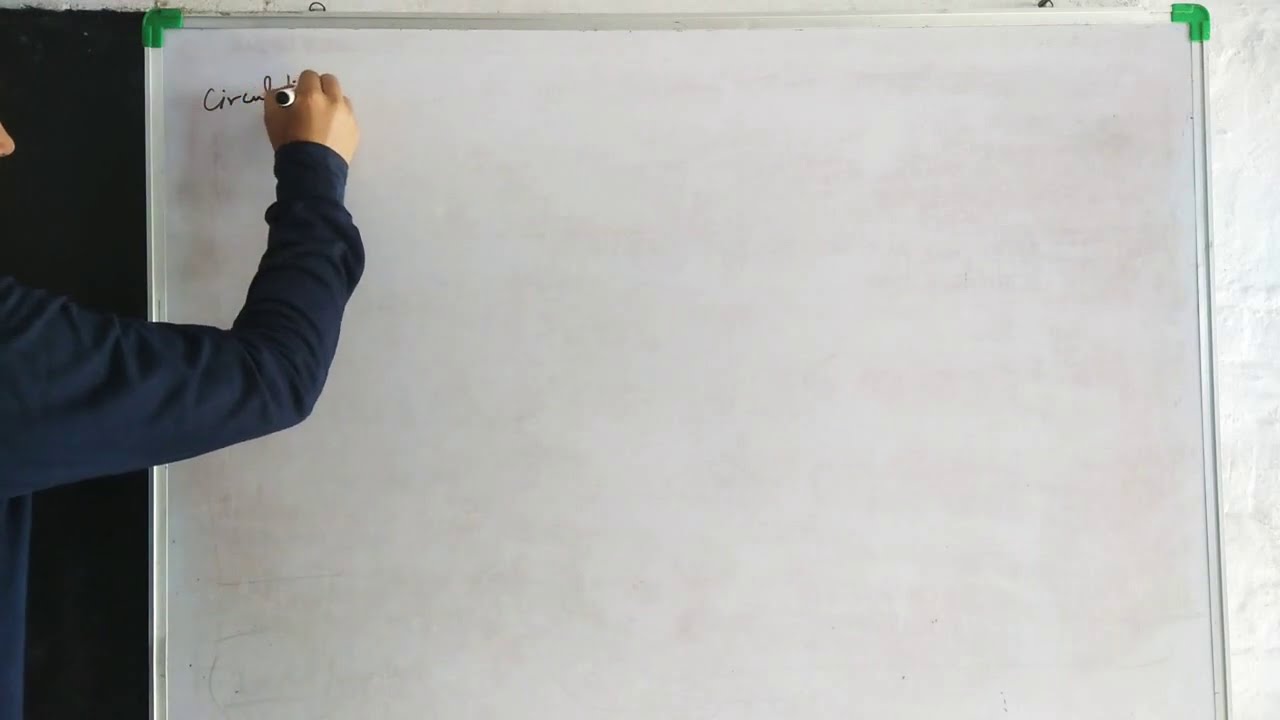The photograph captures a man or person writing on a whiteboard, predominantly filling the frame in landscape orientation. The individual, characterized by an olive skin tone and clad in a long-sleeved navy blue sweatshirt, is partially visible with just their right arm and the tip of their nose peeking into the shot from the left side. They hold a black marker and are in the midst of writing the letters "C-I-R-C-U-L," although the rest of the word is obscured by their hand.

The whiteboard, bordered by silver edges and featuring green tabs fixed at its upper left and right corners, shows signs of heavy use with black smudges from prior markings. Despite being recently erased, remnants of previous writings are still visible. A black border is discernible next to the individual, potentially forming part of the background or frame. The overall scene conveys a focused moment of teaching or presentation activity.